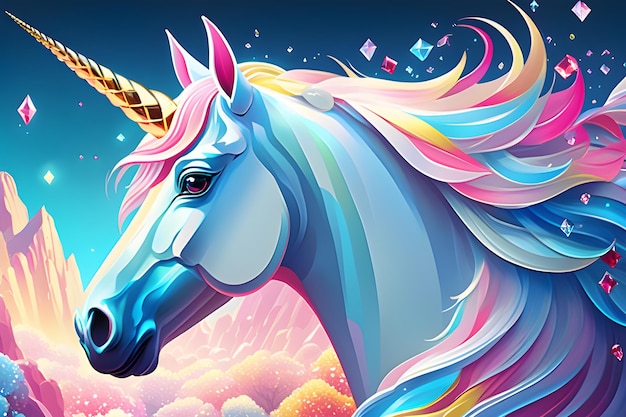The image is a detailed computer-generated artwork of a unicorn, prominently featuring its head and neck in the center. The unicorn is facing toward the left side, with a golden metallic horn stretching out towards the upper left corner of the image. Its nose is positioned at the lower left-hand corner. The unicorn is depicted in a bluish hue with a vibrant, rainbow-colored mane that includes shades of blue, yellow, pink, and purple. Its pointed ears have pink interiors. Surrounding the unicorn are floating diamonds or octahedral gemstones in a variety of colors like blue, purple, and red, set against a night sky filled with magical colors. The background features a whimsical pink and yellow valley with mountainous scenery, completing the fantastical appearance of the scene.